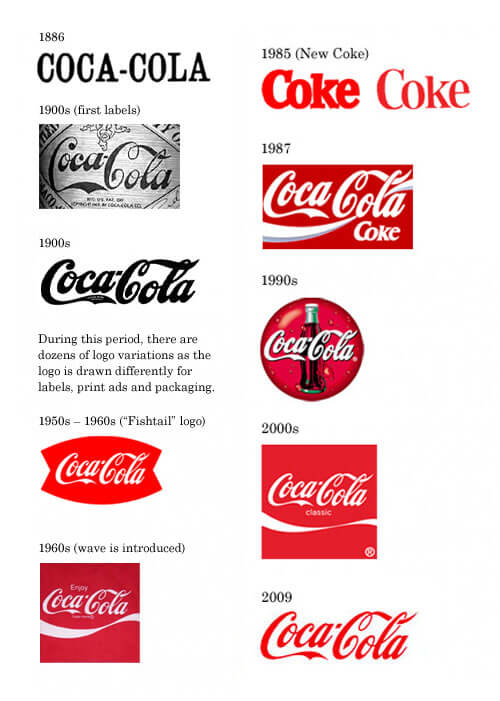This detailed color image showcases the evolution of Coca-Cola logos from 1886 to 2009, arranged in two columns. The left column begins with the logo from 1886, featuring a plain serif font in black. Below it, the 1900s logo introduces a more sophisticated, stylized script font that resembles the modern Coca-Cola logo. The mid-20th century brings further changes; in the 1950s and 1960s, a distinctive red background with white lettering and a fishtail design appears. Across the top of the right column, the 1985 New Coke logo shows a significant shift with red text on a white background. After New Coke's failure, the 1987 logo returns to a style similar to earlier versions. The 1990s logo includes a circular design featuring the iconic Coca-Cola bottle. The 2000s design continues to evolve with a modern wave element, and at the bottom, the 2009 logo revisits the early 1900s style but with a red font. Each logo reflects the brand's continuous adaptation and historical milestones.